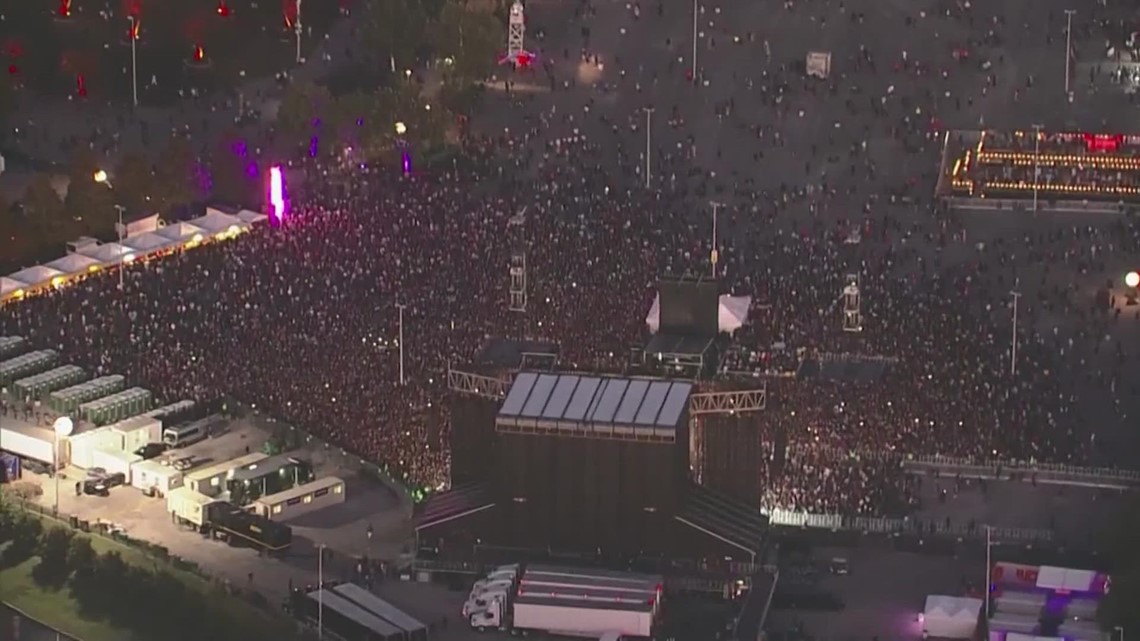An aerial photograph taken at night, possibly by a drone, captures a massive, densely-packed event, likely a concert, in a large urban space. The focal point is a stage with a large black structure and towering staging frames, viewed from behind. The surrounding area is filled with semi-trailer trucks, suggesting a large-scale setup. The photograph, dimly lit due to the nighttime setting, reveals a sea of people standing shoulder-to-shoulder, densely populating an area that spans several acres. The scene is characterized by dim and scattered lighting, including a notable pink light on the left and a significant red light in the center. Raindrops are visible, indicating that the photograph was taken during a rainy night. Tall buildings and possibly a stadium are discernible in the background, adding to the urban concert atmosphere.